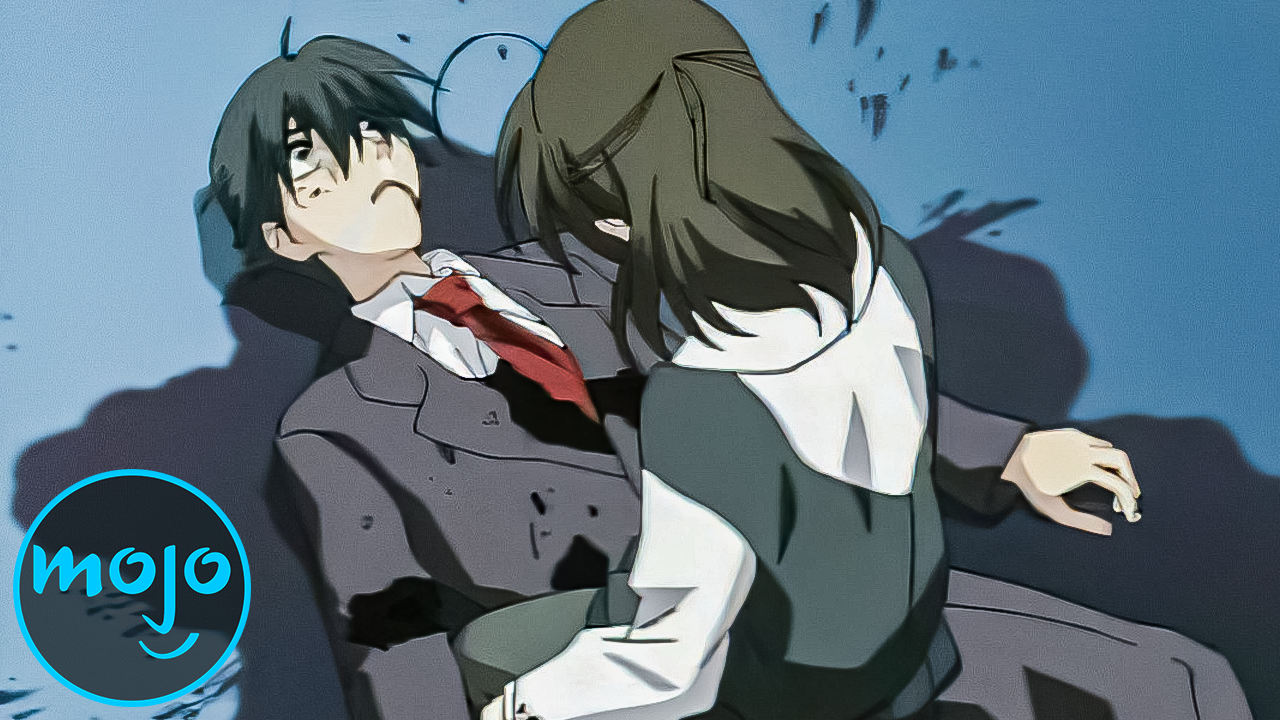In this anime-style illustration, a young man lies motionless on the ground, clad in a gray suit with a red tie and white shirt. His long, dark hair partially obscures his face, which is smeared with blood while his unblinking eyes stare skyward. A shadow enhances the drama of the scene, extending from the man's body. Beside him, a young girl with short hair and a gray frock over a white shirt kneels, her face turned away as she tries to wake him. The backdrop transitions from lighter to darker shades of blue, creating a somber atmosphere. In the bottom left corner, the "Mojo" logo appears in a bluish-green circle, adding a distinctive touch to the illustration.